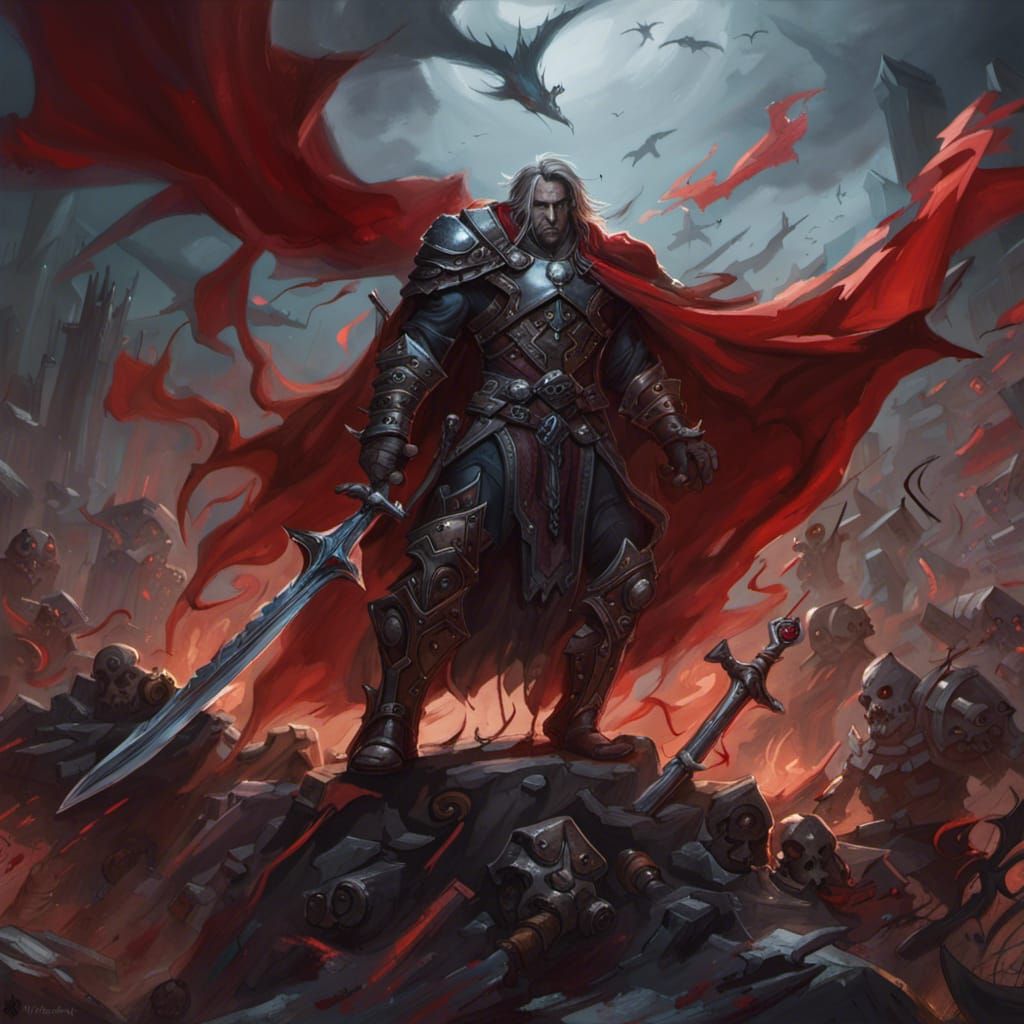In the center of this fantasy-themed artwork, a stern, pale-faced man with long gray hair stands defiantly atop a rock. He is heavily armored, with intricate metal plating on his shoulders, chest, and gloves, and wields a large sword in his right hand. His tattered, vibrant red cape billows dramatically in contrast to the darker, gothic tones of black, dark blue, and gray that dominate the scene. At the base of the rock lies another sword, partially embedded and dented. Surrounding this central figure are several menacing mutant-like soldiers and skeletal creatures, particularly noticeable on the left and right sides of the image. Above, the sky is filled with flying dragon-like creatures, adding an eerie sense of fantasy and danger to the composition.